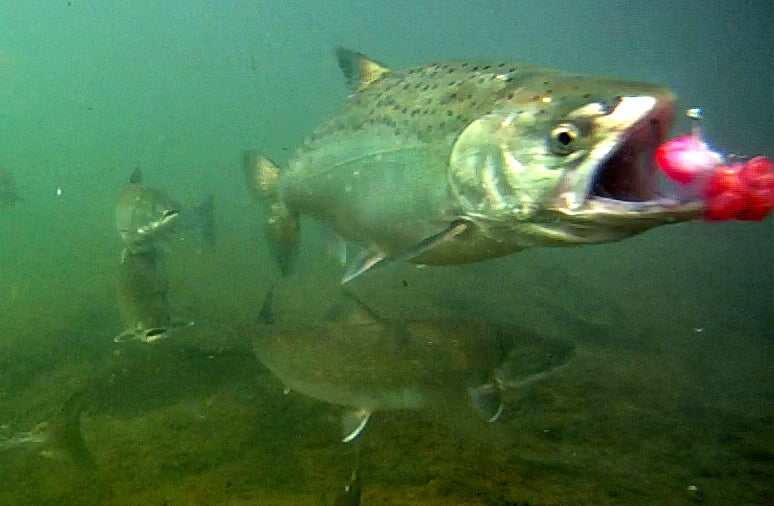This detailed underwater photograph vividly captures a tense moment in the aquatic world, featuring an array of fish, primarily likely trout. At the center of the action, a large trout dominates the foreground, mouth wide open, eagerly approaching a tantalizing red lure that resembles a bulbous creature or perhaps a piece of bait entailing the innards of another fish. The scene unfolds in murky, greenish-brown water at the bottom of a riverbed, where sediment and poor visibility hint at a natural yet somewhat polluted environment. Surrounding this central fish, three other trout watch in apparent horror, their silver bodies with distinctive black speckles subtly illuminated amidst the gloomy water. One fish to the left, slightly elevated, and two on the right, one swimming near the riverbed and the other higher up, create a dynamic composition, emphasizing the drama and imminent danger in this compelling underwater action shot.